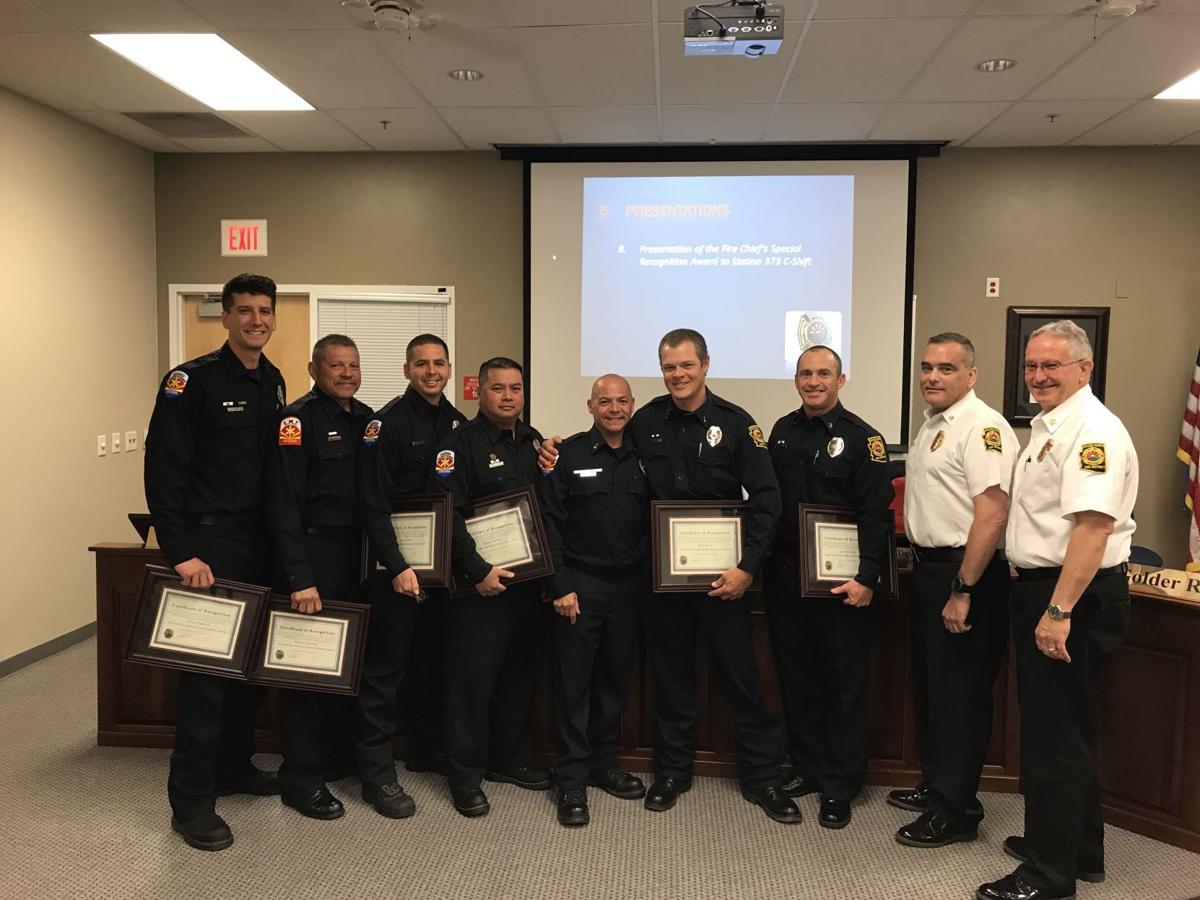In this image, a group of seven men is standing in a formal setting that resembles a city hall or a police station. These men are uniformed officers, six of whom are dressed in very dark navy or black attire, while the two on the far right are wearing white shirts with dark pants, possibly indicating higher ranks or different roles. Each of the officers in dark uniforms is holding a framed certificate or award, identifiable by a visible seal in the corner of each frame. In the background, an overhead projector and a screen display a PowerPoint slide with indistinct writing, adding to the official atmosphere. An American flag is positioned on the back right side of the room, and an open exit door is visible to the left. The setting features typical ceiling panels with long halogen lights, reinforcing the institutional ambiance. The group is positioned in front of a large desk, partially visible behind them.